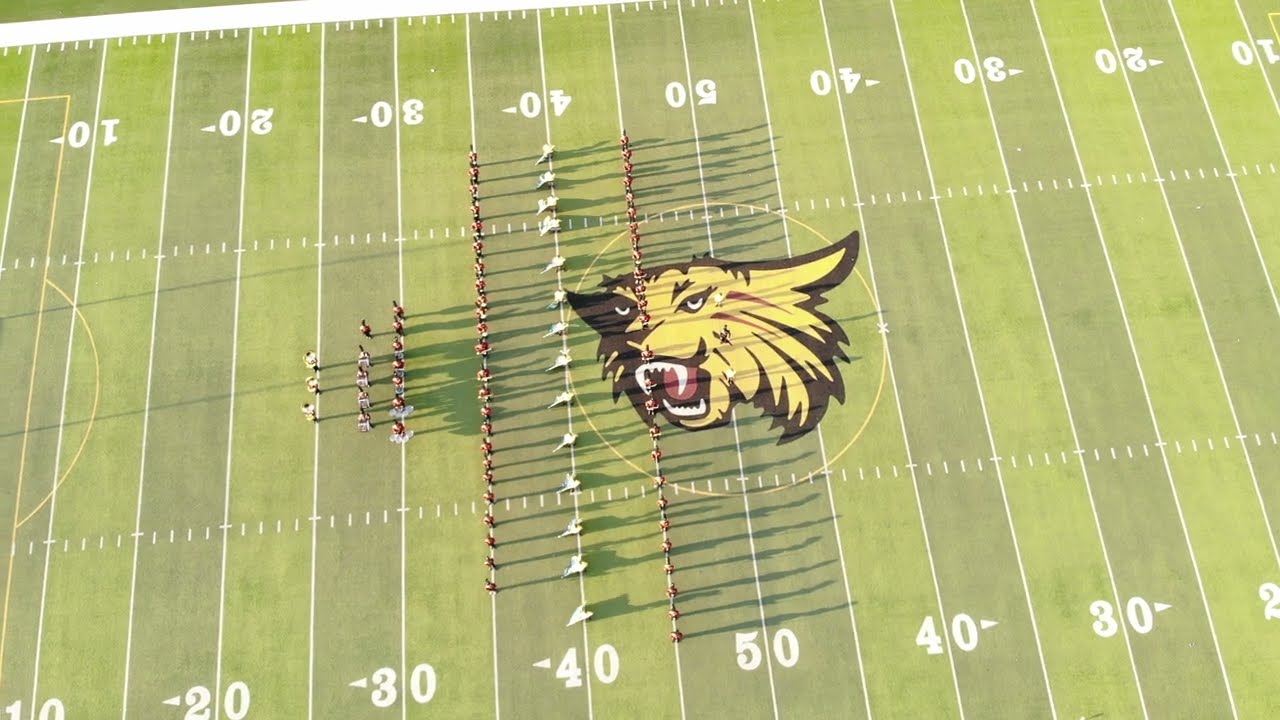The image is an overhead, aerial photo of an American football field filled with vibrant colors and details. At the center of the field is a distinct logo resembling a cat, suggesting it may belong to a lesser-known team or institution. The scene is set outdoors, likely in the middle of the day, as indicated by the bright lighting. The band appears to be performing on the field, organized in several rows of varying lengths and positioned across different yard lines. Notably, a group lines up on the 50-yard line, another long row stretches along the 45, a white-colored line is situated on the 40, followed by another line on the 35, a smaller line on the 30, and three individuals stand on the 25. Additional members are distributed around the 27-yard line. The football field's surface displays alternating bands of color, including shades of green, orange-red, yellow, black, and white, contributing to the overall vividness of the image.